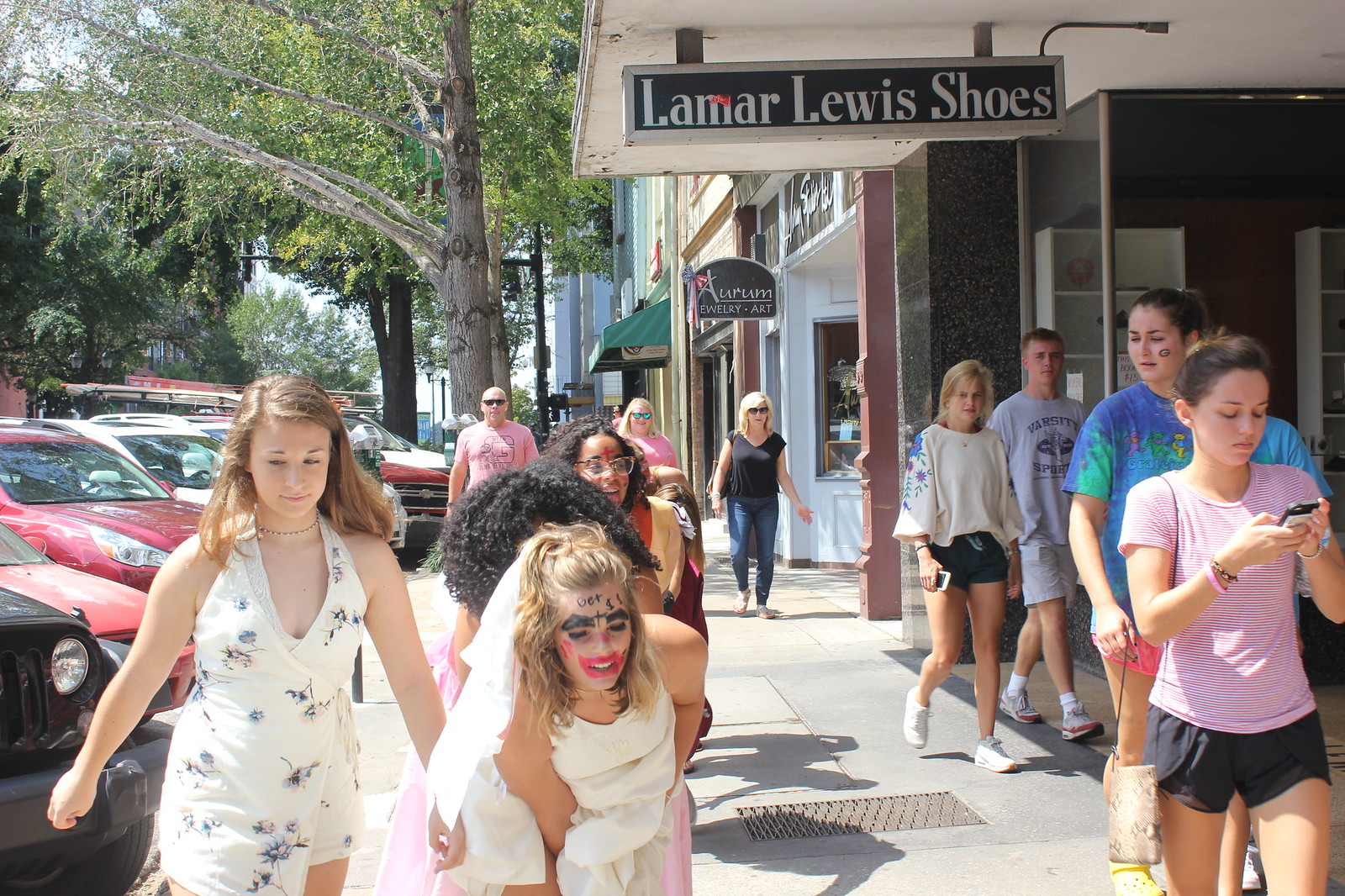The image shows a bustling downtown street scene at a busy shopping center, with rows of shops and clusters of people walking along the sidewalk. On the right side, signs for "Lamar Lewis Shoes" and "Oram Jewelry and Art" are visible above the shops, while several parked cars line the street to the left. A diverse group of around 10 people is seen, including some older individuals walking in the background. 

Among them, a striking figure at the forefront catches the eye: a woman in an exaggerated wedding ensemble, featuring a veil and what appears to be a parody of bridal attire. Her face is heavily made-up with exaggerated, clown-like makeup; lipstick is smeared well beyond her lips, eyebrows appear to be dark and drawn on with thick, sharpie-like strokes, and "G.E.T." is scribbled on her forehead. A red smudge marks her nose, and she wears a short, floral halter neck dress. Behind her, a woman with curly black hair seemingly supports her by holding up her dress. Another woman nearby is conspicuously absorbed in her phone. Trees dot the sidewalk, adding a touch of greenery to the urban setting.